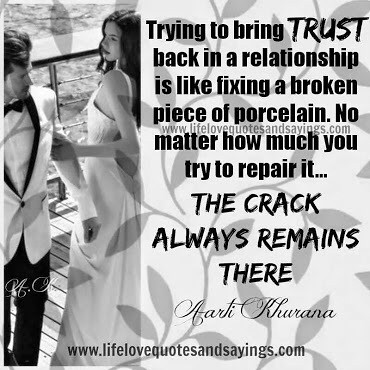This black and white photo features a woman in a wedding dress tightly grasping a man's arm; he is dressed in a white wedding suit, suggesting both individuals are likely models. The background is adorned with a light gray leaf pattern that subtly frames the black text overlay. The image is accompanied by an inspirational quote which reads, "Trying to bring trust back in a relationship is like fixing a broken piece of porcelain. No matter how much you try to repair it, the crack always remains there." This poignant message is credited to Arti Kurana, although the cursive signature is somewhat indistinct. Below the quote, the website www.lifelovequotesandsayings.com is clearly displayed. The left side of the image presents the couple standing together, possibly on a dock or a boat, adding to the romantic yet introspective feel of the composition.